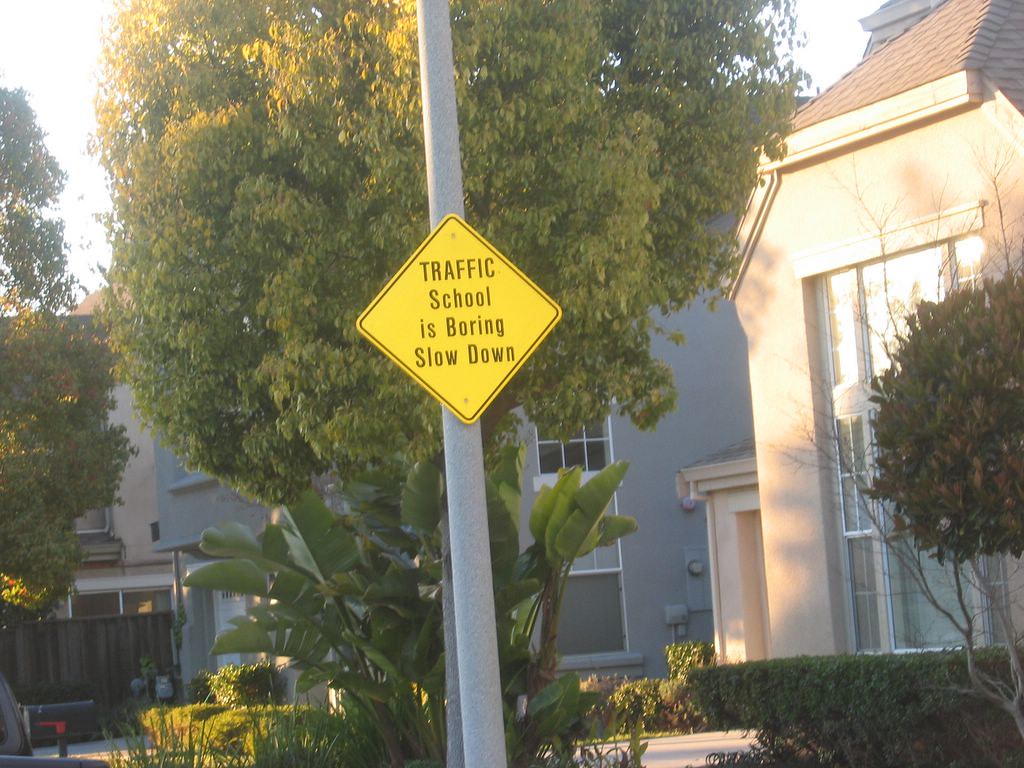In the center of the image stands a silver pole with a diamond-shaped, yellow street sign bordered in black, bearing the message "Traffic school is boring, slow down" in black lettering. Dominating the background is a large tree, its expansive canopy taking up much of the picture, with a smaller tree situated just below it. To the side, there are several bushes and a mailbox featuring a red flag. Part of a car is visible near the gas meter situated in the left-hand corner, adjacent to a white garage door of a gray house. This gray house also showcases two windows and an electric meter mounted on its exterior. 

To the right of the gray house, there is another house in a whitish-tan hue. This neighboring house features a large front window and is partially obscured by a substantial bush and a tree. Further details include another tan house next to the gray one, with just the top of its sliding doors and a small part of a window visible due to a wooden fence and a large tree in the foreground. Sunlight reflects off the whitish-tan house on the right, illuminating the scene.